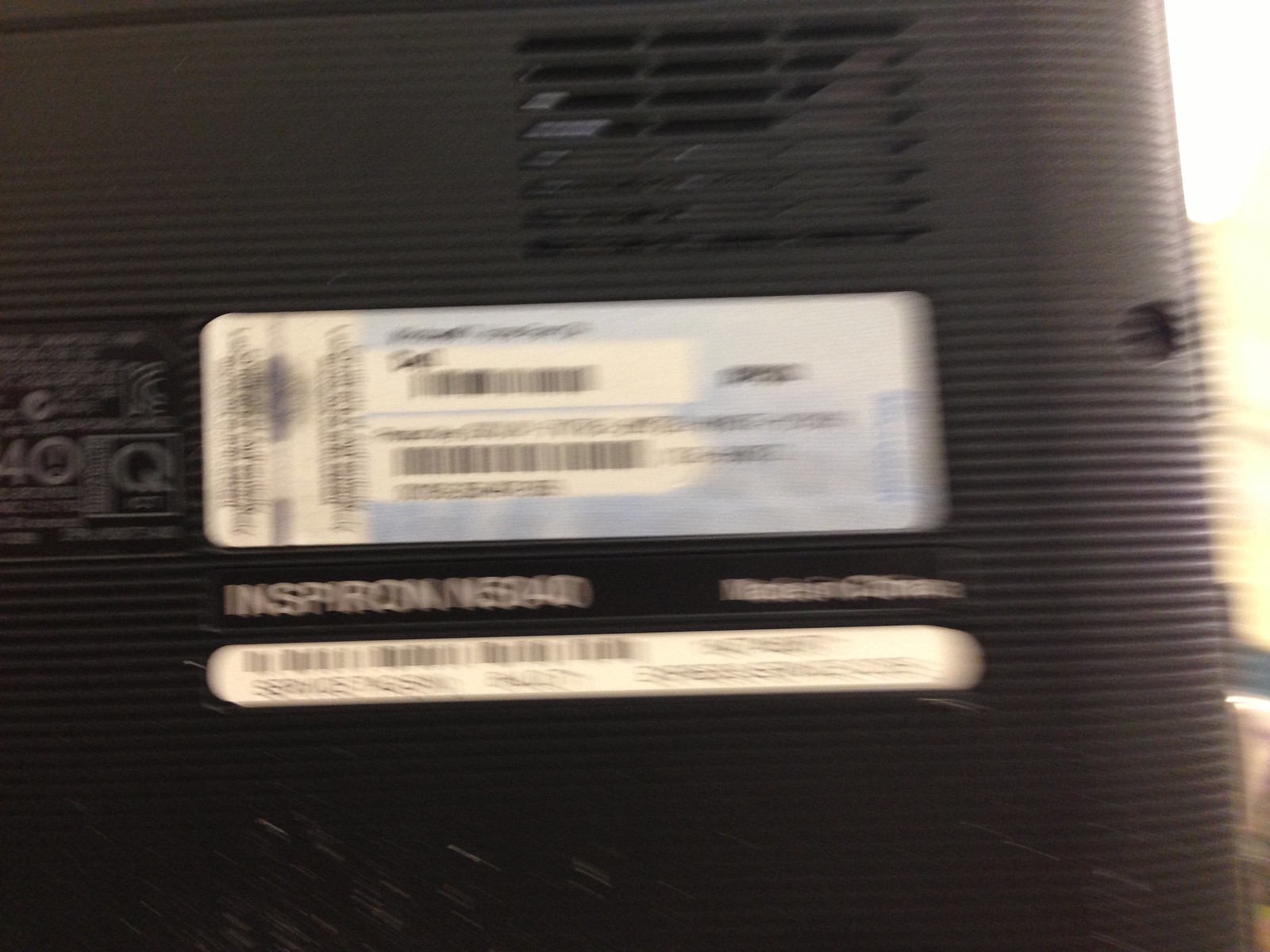The image captures a blurry close-up of the back panel of a black electronic device, possibly a laptop or monitor. The surface is predominantly black with a series of horizontal ridges running across it. The central area of the panel is made of plastic, where a rectangular sticker is prominently displayed. This sticker has a light blue border and a white interior, featuring two barcodes: a smaller one on top and a slightly larger one at the bottom. Both barcodes are in the standard black-and-white format. Surrounding these barcodes is various product information printed in black text. Beneath the sticker, additional text is visible, including the word "Spartan" and an indication that the device is "Made in China."